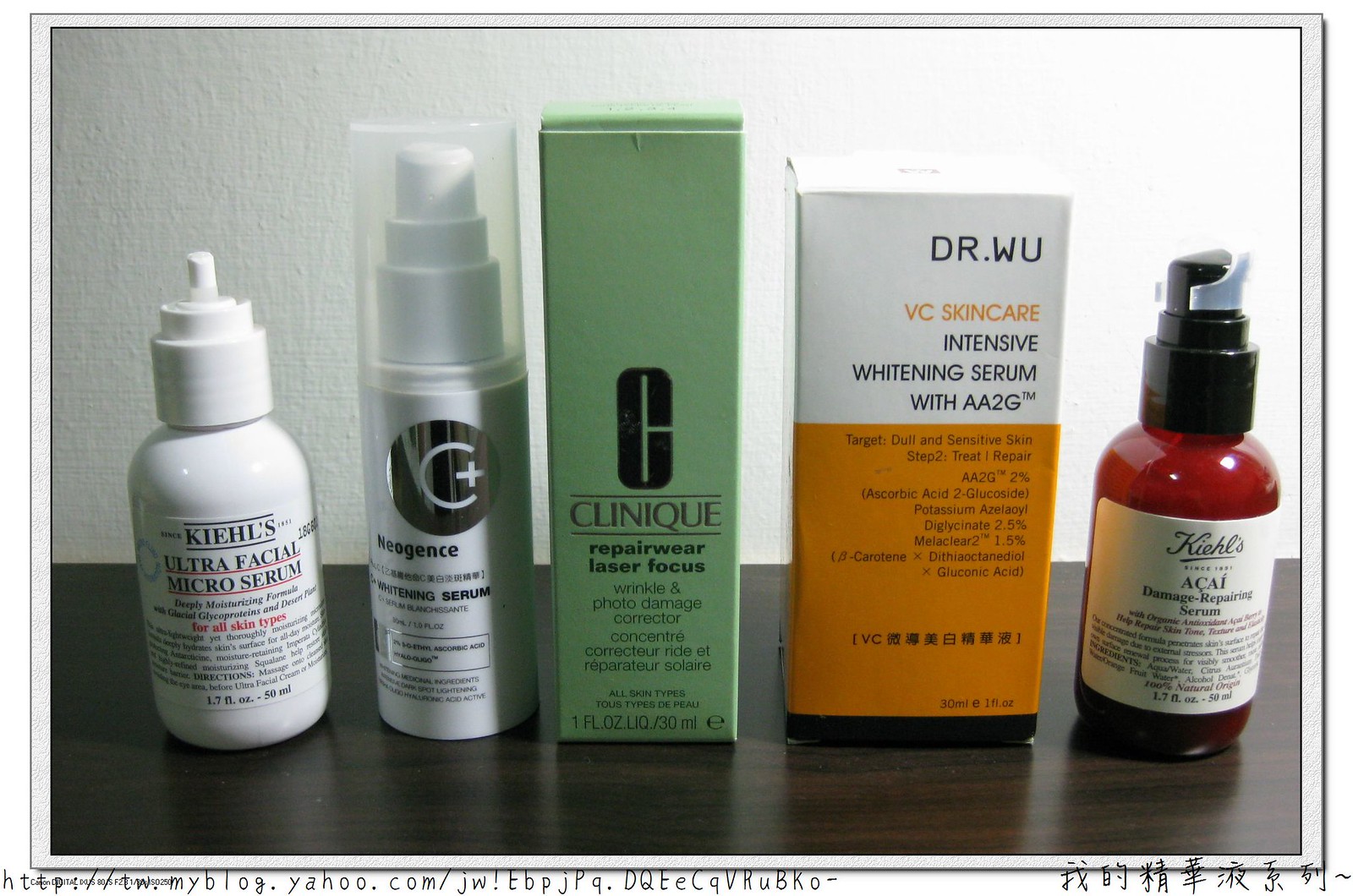The image features five distinct skincare items placed on a brown table against a white wall backdrop. 

1. The first item is Kiehl's Ultra Facial Micro Serum, presented in a sleek white plastic bottle.
2. Next is a product from Neogence, also housed in a white container, notable for its spray top which is protected by a see-through cap. The label prominently displays a silver circle with a "C+" symbol and identifies the product as a whitening serum.
3. The third item is a green box labeled Clinique Repairwear Laser Focus Wrinkle & Photo Damage Corrector. The box is light green and features a large "C" above the word "Clinique."
4. Fourth is a box with a gold and white design from Dr. Wu, branded as VC Skincare Intensive Whitening Serum with AA2G. It targets dull and sensitive skin and details the treatment steps, percentage concentrations, and ingredients.
5. Lastly, there is a brown glass bottle from Kiehl's, titled Acai Damage Repair Serum. This bottle has a black spray top protected by a white cap.

Each product is carefully labeled with its respective quantities in fluid ounces. The overall arrangement is neat, showcasing the variety of skincare solutions available.